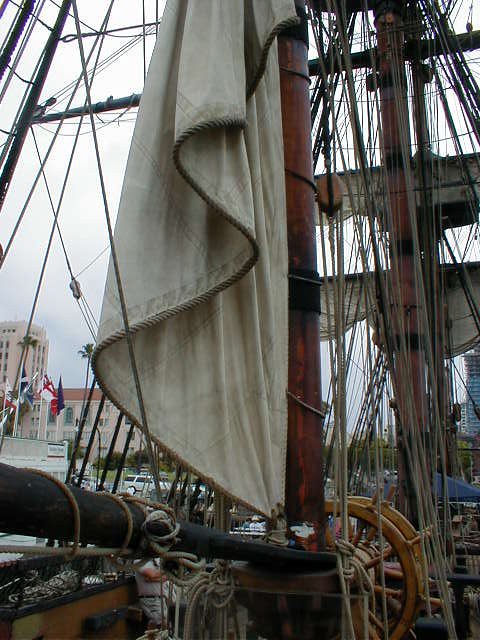The image captures an intriguing scene of a city harbor dominated by an old-style sailboat, reminiscent of a pirate ship. The foreground showcases the boat's wooden steering wheel with classic spoked design, numerous ropes, and weathered sails supported by tall masts. The vantage point appears to be from the deck of the ship, as the intricate details of the ship's mechanism and deck rigging are visible. The background reveals a modern cityscape with various buildings, including a distinctive blue skyscraper, possibly a condo building, and a brown building with a brown roof, beside which an SUV is parked, adding to the American urban ambiance. The gray, overcast sky suggests a cloudy day, and several flags can be seen, possibly attached to a hotel or another prominent building, enhancing the scene with a mix of historical and contemporary elements.